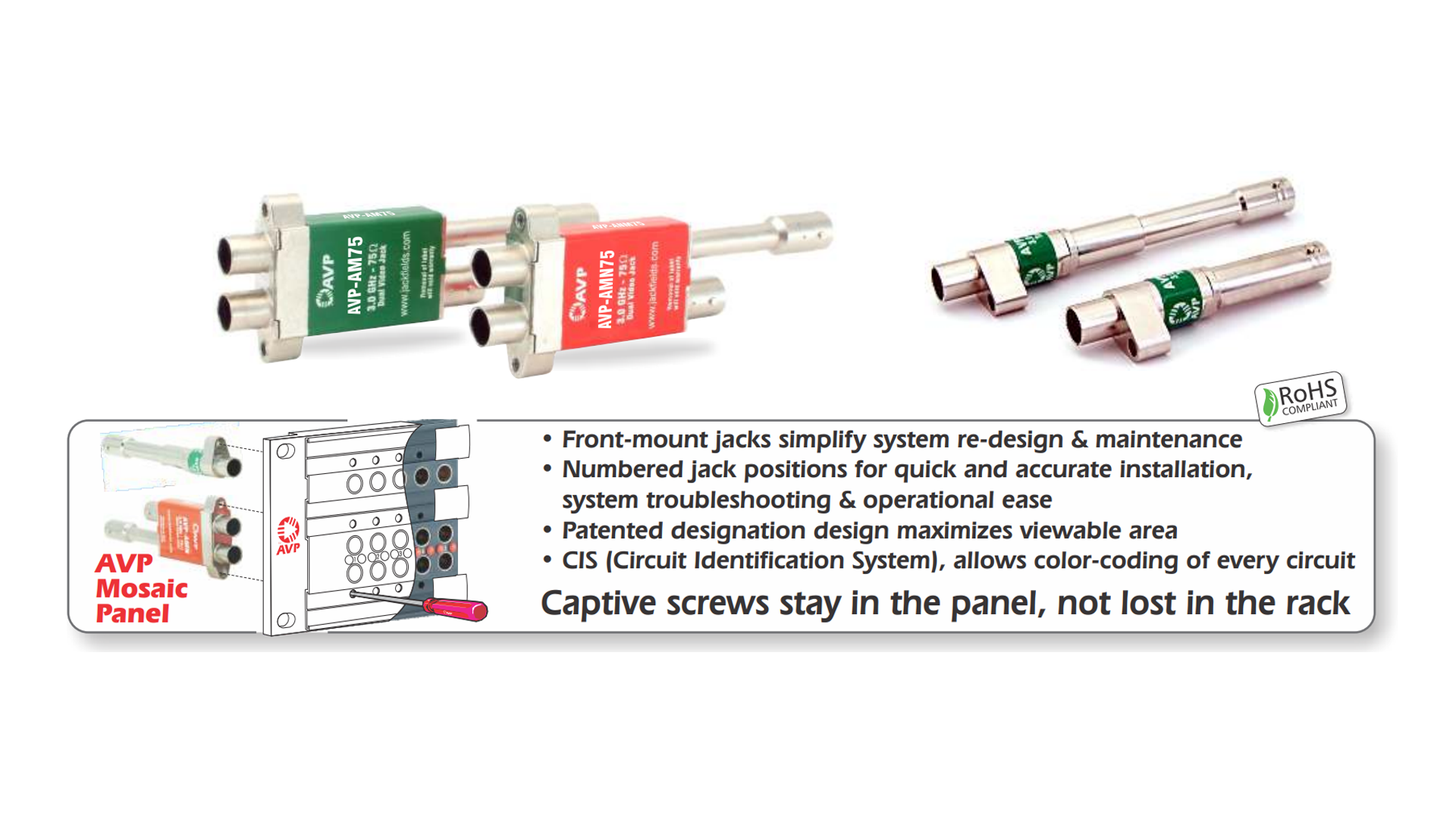The image is an advertisement for an AVP Mosaic Panel, which features various front-mounted jacks and screws designed for AV equipment. The panel showcases multiple jacks in different sizes, with distinct red and green labels for easy identification. The bottom section of the image includes a detailed text box with a slim black border, featuring crucial product features: "Front Mounted Jack Simplify System Redesign and Maintenance," "Numbered Jack Positions for Quick and Accurate Installation, System Troubleshooting, and Operational Ease," "Patented Design Maximizes Viewable Area," and "CIS Circuit Identification System Allows Color Coding of Every Circuit." Additionally, it emphasizes that "Captive Screws Stay in the Panel, Not Lost in the Rack." The entire advertisement is set against a plain white background, and it includes a small diagram next to the red text reading "AVP Mosaic Panel."